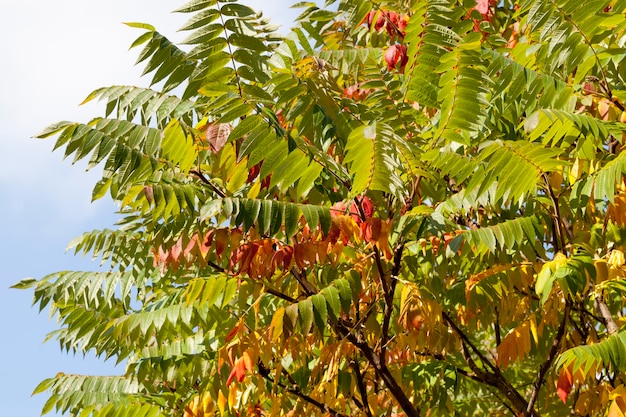The outdoor image captures an exotic tree that dominates the majority of the frame. Displaying a diverse array of colors, the tree has leaves that are primarily a bright green, interspersed with vivid yellow, rich brown, and deep red hues. The tree's slender, dark brown branches—some almost black—extend outward, creating a sense of bilateral symmetry with leaves radiating from either side, reminiscent of a fern yet uniformly elongated. A fragment of a clear blue sky and a partial white cloud can be seen in the background, adding to the early fall atmosphere of the scene. The image is devoid of text and people, focusing exclusively on this vibrant tree with its striking, mixed foliage, and intricate branching pattern.